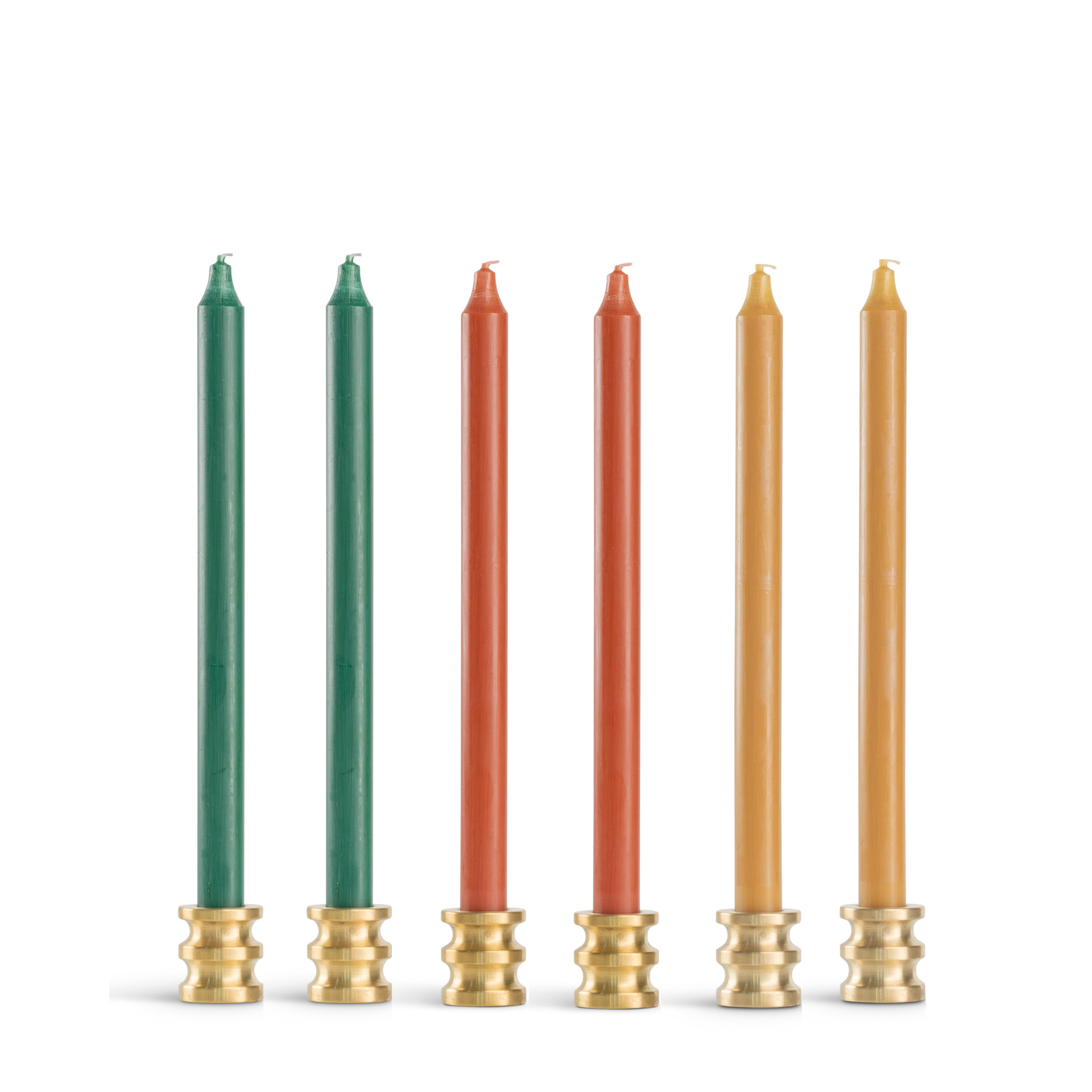This image showcases six tall, thin, tapered candles elegantly arranged against an all-white background. The candles are organized by color: the first two on the left are a rich evergreen, the middle two are a light red, and the two on the right are a golden yellowish-orange, almost an amber hue. Each candle is unburnt with a pristine white wick at the top. They are uniformly placed in identical round, brass candle holders that feature a distinctive design with two indented grooves encircling them, creating a barrel-shaped appearance. The consistent size and placement of these candles, coupled with the minimalist background, highlight their vivid colors and sophisticated holders without any additional distractions or text.